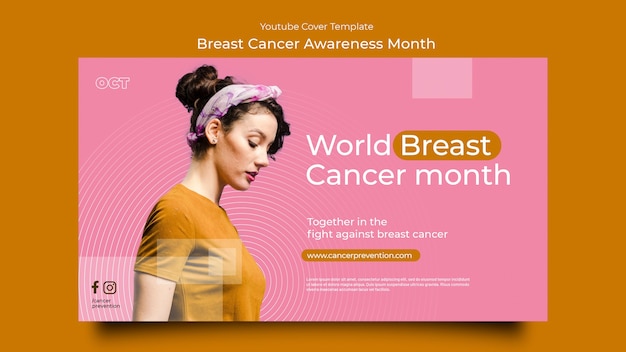This image features an orange background with a prominent white text that reads "YouTube Cover Template" about three lines down from the top. Beneath this, larger white letters announce "Breast Cancer Awareness Month." Lower down on the image, there's a pink rectangle on the left side, showcasing a profile of a woman with dark hair in a bun, wearing a scarf and an orange short-sleeved top. Soft white lines radiate from around her head and chest, creating a bullseye effect. 

To the right of the woman's profile, aligned with her forehead, bold white letters state "World Breast," where the word "Breast" has an orange oval behind it. Below this, "Cancer Month" is printed in white letters. Further down, about four lines below, the message "Together in the Fight Against Breast Cancer" is displayed in white text. An oval button containing a website URL is placed below this message, followed by three lines of fine white print at the bottom of the image.